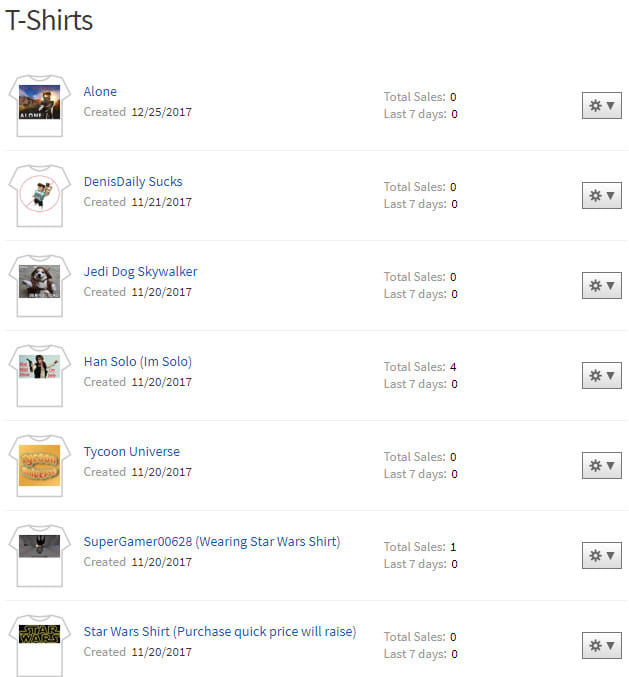This image features a detailed list of t-shirt options set against a white background. At the very top left corner, the word "T-Shirts" is prominently displayed in large, light black font. The list consists of 7 rows, each representing a different t-shirt design.

- Row 1: 
  - Image: Picture of the t-shirt on the left
  - Name: "Alone" (in blue font)
  - Additional Info: "Total Sales" and "Last 7 Days" displayed towards the right, with a settings button at the far right
  - Created Date: Displayed below the t-shirt name

- Row 2: 
  - Image: Picture of the t-shirt on the left
  - Name: "Dennis Daily Sucks" (in blue font)
  - Additional Info: "Total Sales" and "Last 7 Days" displayed towards the right, with a settings button at the far right
  - Created Date: Displayed below the t-shirt name

- Row 3: 
  - Image: Picture of the t-shirt on the left
  - Name: "Jedi Dog Skywalker" (in blue font)
  - Additional Info: "Total Sales" and "Last 7 Days" displayed towards the right, with a settings button at the far right
  - Created Date: Displayed below the t-shirt name

- Row 4: 
  - Image: Picture of the t-shirt on the left
  - Name: "Han Solo I'm Solo" (in blue font)
  - Additional Info: "Total Sales" and "Last 7 Days" displayed towards the right, with a settings button at the far right
  - Created Date: Displayed below the t-shirt name

- Row 5: 
  - Image: Picture of the t-shirt on the left
  - Name: "Tycoon Universe" (in blue font)
  - Additional Info: "Total Sales" and "Last 7 Days" displayed towards the right, with a settings button at the far right
  - Created Date: Displayed below the t-shirt name

- Row 6: 
  - Image: Picture of the t-shirt on the left
  - Name: "Super Gamer 00628 wearing Star Wars shirt" (in blue font)
  - Additional Info: "Total Sales" and "Last 7 Days" displayed towards the right, with a settings button at the far right
  - Created Date: Displayed below the t-shirt name

- Row 7: 
  - Image: Picture of the t-shirt on the left
  - Name: "Star Wars shirt. Purchase quick, price will raise" (in blue font)
  - Additional Info: "Total Sales" and "Last 7 Days" displayed towards the right, with a settings button at the far right
  - Created Date: Displayed below the t-shirt name

All information is presented in gray or black font, except for the names of the t-shirts, which are in blue. The settings button appears consistently at the far right of each row, providing additional management options for each t-shirt listed.